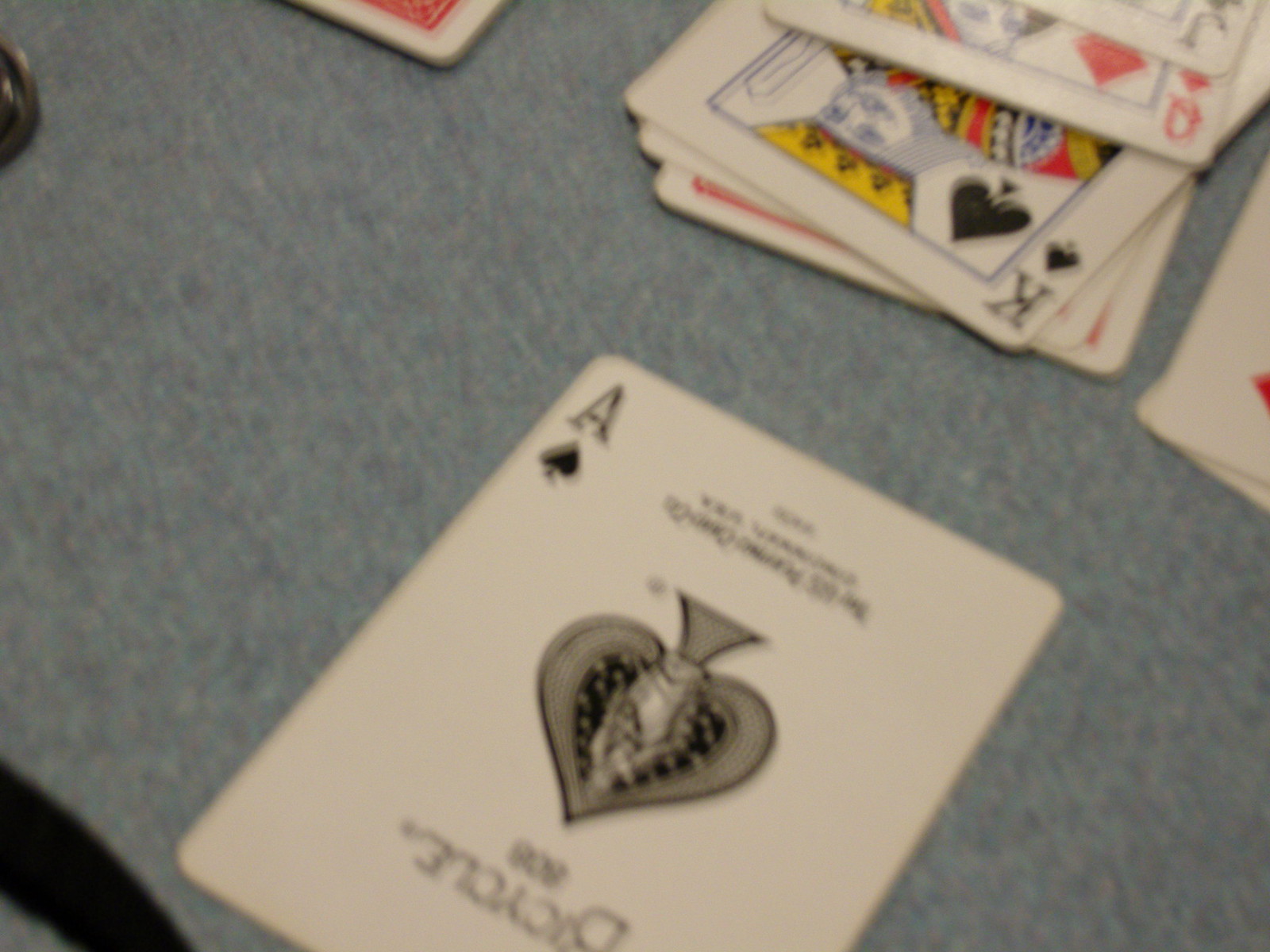This image showcases a meticulously arranged collection of playing cards set against a light blue surface, focusing predominantly on the Ace of Spades card. 

The primary card, the Ace of Spades, takes center stage. Its white background prominently features the letter 'A' and a black spade symbol in the top left corner. Dominating the center of the card is a large, intricately designed spade, shaded with delicate lines and adorned with white dots. There is black text underneath the central spade, though it's partially obscured and not fully legible.

Surrounding the Ace of Spades are additional playing cards. In the top right corner, a portion of a Jack card (marked 'J' in black) is visible, though it appears to be sheared off at the edge. Below it is the Queen of Diamonds, recognizable by the red diamond symbol and the letter 'Q'. There is also an object displaying a mix of colors—white, black, blue, red, and yellow—though its nature is unclear in the context.

Beneath these cards lies the King of Spades, featuring the black spade symbol and a finely detailed image of a king. The king is adorned with a yellow crown and has facial features drawn in blue. His opulent jacket is a patchwork of yellow, red, black, white, and blue, all accentuated by clear outlining.

The reverse sides of some of the cards are also visible, characterized by a patterned red and white backing. The entire scene is set atop a smooth, light blue surface, providing a serene backdrop to the vivid details of the playing cards.